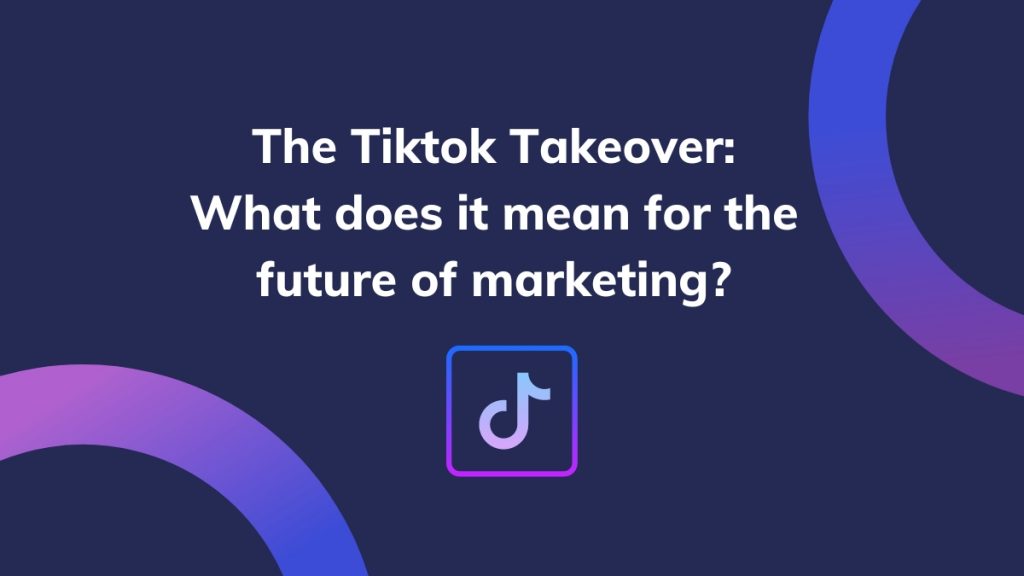A computer screen displays a visually engaging banner with a deep purple background. The headline in bold, white text reads: "The TikTok Takeover: What Does It Mean for the Future of Marketing?" This heading suggests a focus on an upcoming talk or webinar aimed at exploring the implications of TikTok on modern marketing strategies.

Centralized below the text is the iconic TikTok logo, a stylized music note encapsulated within a square. The square features an ombre gradient that shifts from vibrant pink to soothing blue, echoing the trendiness of the TikTok brand.

Adding visual interest, the design includes two quarter-circle outlines: one in the bottom left corner and another in the top right corner of the banner. These curves also feature a pink-to-blue ombre gradient, seamlessly blending with the calming yet dynamic color scheme of the overall design. The harmonious color palette and structured layout work together to create a captivating invitation to the forthcoming event focused on the future of marketing in the TikTok era.